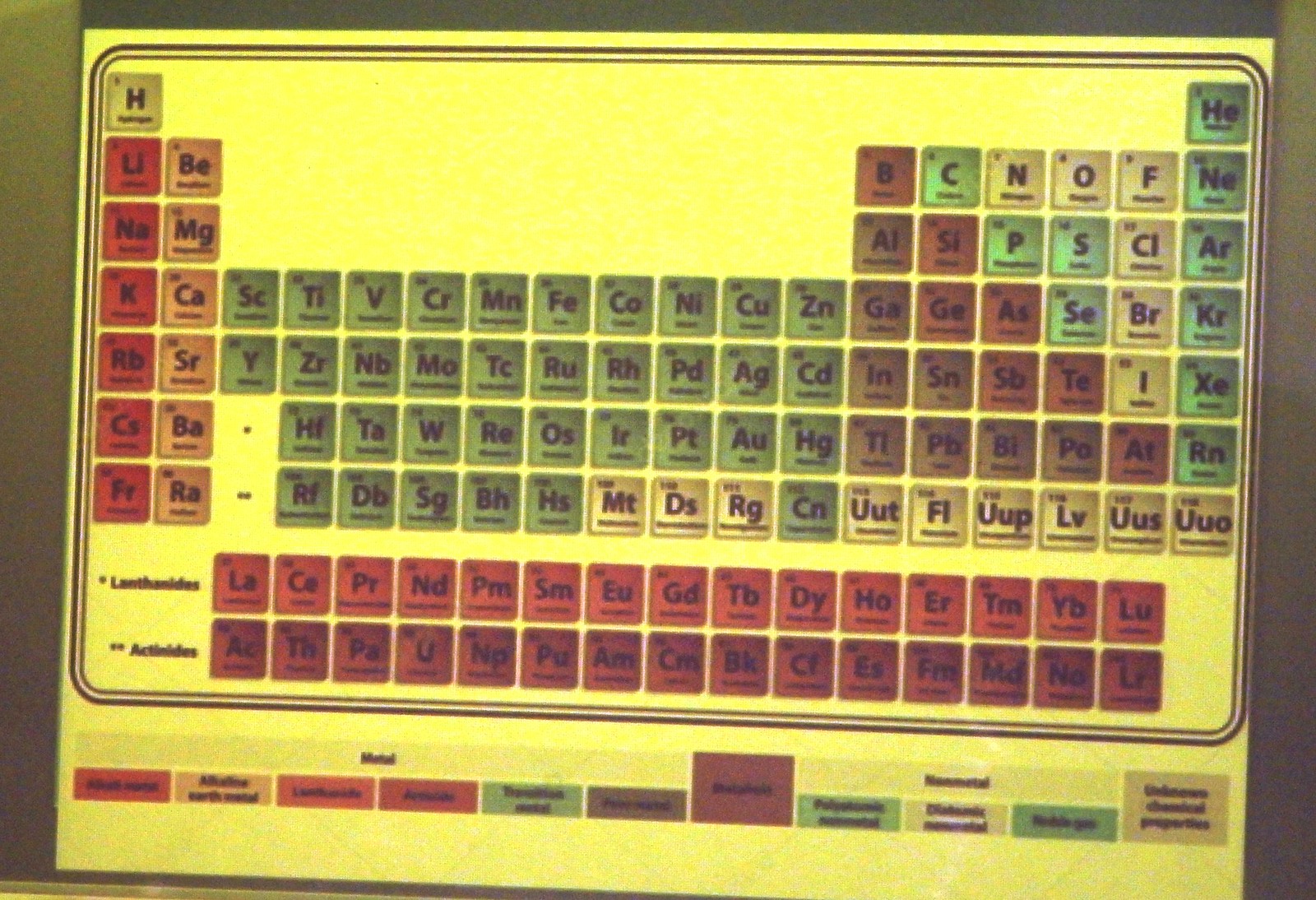The image portrays a slightly askew and somewhat blurry poster of the periodic table of elements, most likely displayed on a wall or a desk, set against a yellow background. Each element is depicted in a color-coded rectangle, with various colors such as yellow, red, orange, green, brown, a burnt orange, darker green, lighter green, pinkish, and purple, indicating different categories like metals and non-metals as outlined in the legend at the bottom of the poster. Specific elements are visible, starting from the upper left with hydrogen (H, in a darker yellow rectangle with black text) and helium (He) proceeding across, then lithium (Li), beryllium (Be), boron (B), carbon (C), nitrogen (N), oxygen (O), fluorine (F), and so forth. Notable elements like sodium (Na), magnesium (Mg), aluminum (Al), silicon (Si), phosphorus (P), sulfur (S), chlorine (Cl), and argon (Ar) are also discernible across their respective rows. The poster includes some notes and a color-coded legend at the bottom, explaining the significance of each color pertaining to the elements, though the exact details are difficult to make out due to the blurriness.